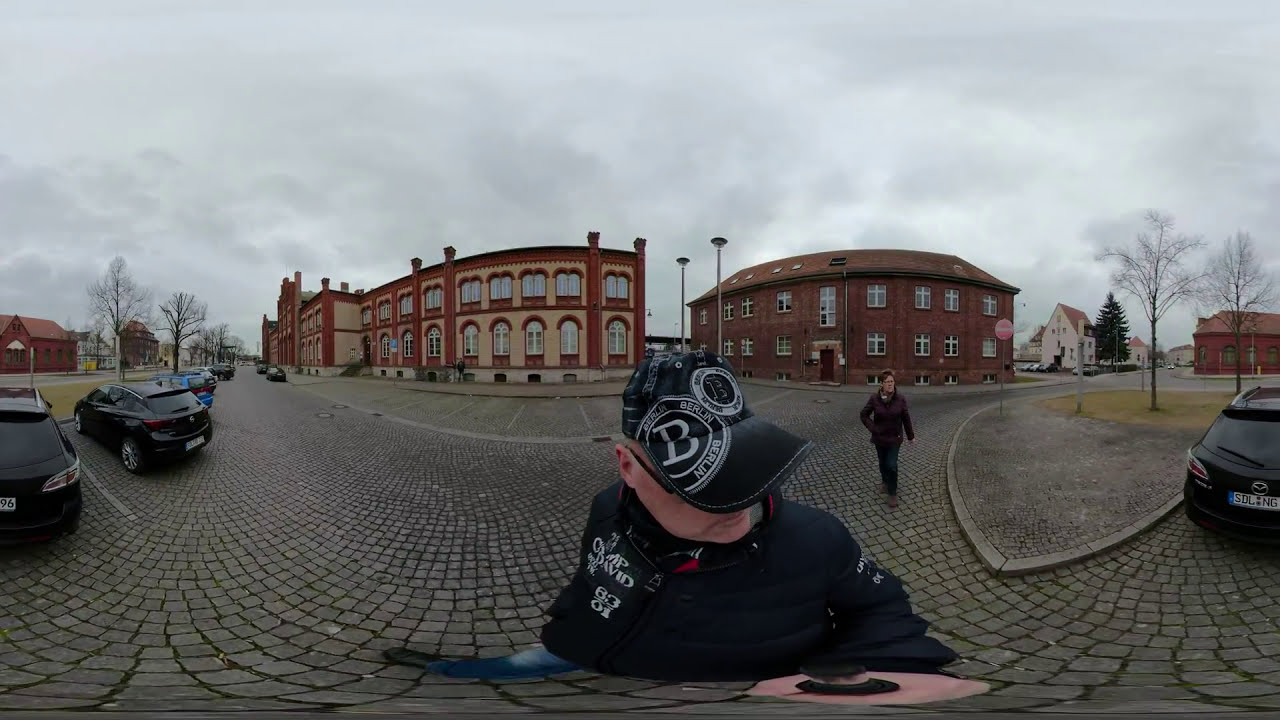The image depicts a bustling urban scene with a focus on a man in the foreground, who is engaging in panoramic photography using a selfie stick. The man, dressed entirely in black with a distinctive black hat marked by a large letter 'B' circled and repeating the word "Berlin" three times, is captured mid-step on a cobblestone street. His jacket, slightly crunched and bearing the name "David" along with the numbers "8301" in two lines, partially hides additional text. 

Behind him, a woman in a purple jacket and black pants is also walking in the same direction, appearing to glance towards the man. To their right, a black car with a European license plate is parked. The left side of the scene is filled with a parking lot that has multiple cars, including black and blue ones arranged in neat rows. The background is dominated by brown and red multi-story buildings, some featuring white trim around their window sections, typical of European architecture. The sky overhead is gray and cloudy, indicating winter, and the bare trees confirm the cold season. Street signs add to the urban setting, enhancing the image's overall European street-side atmosphere.